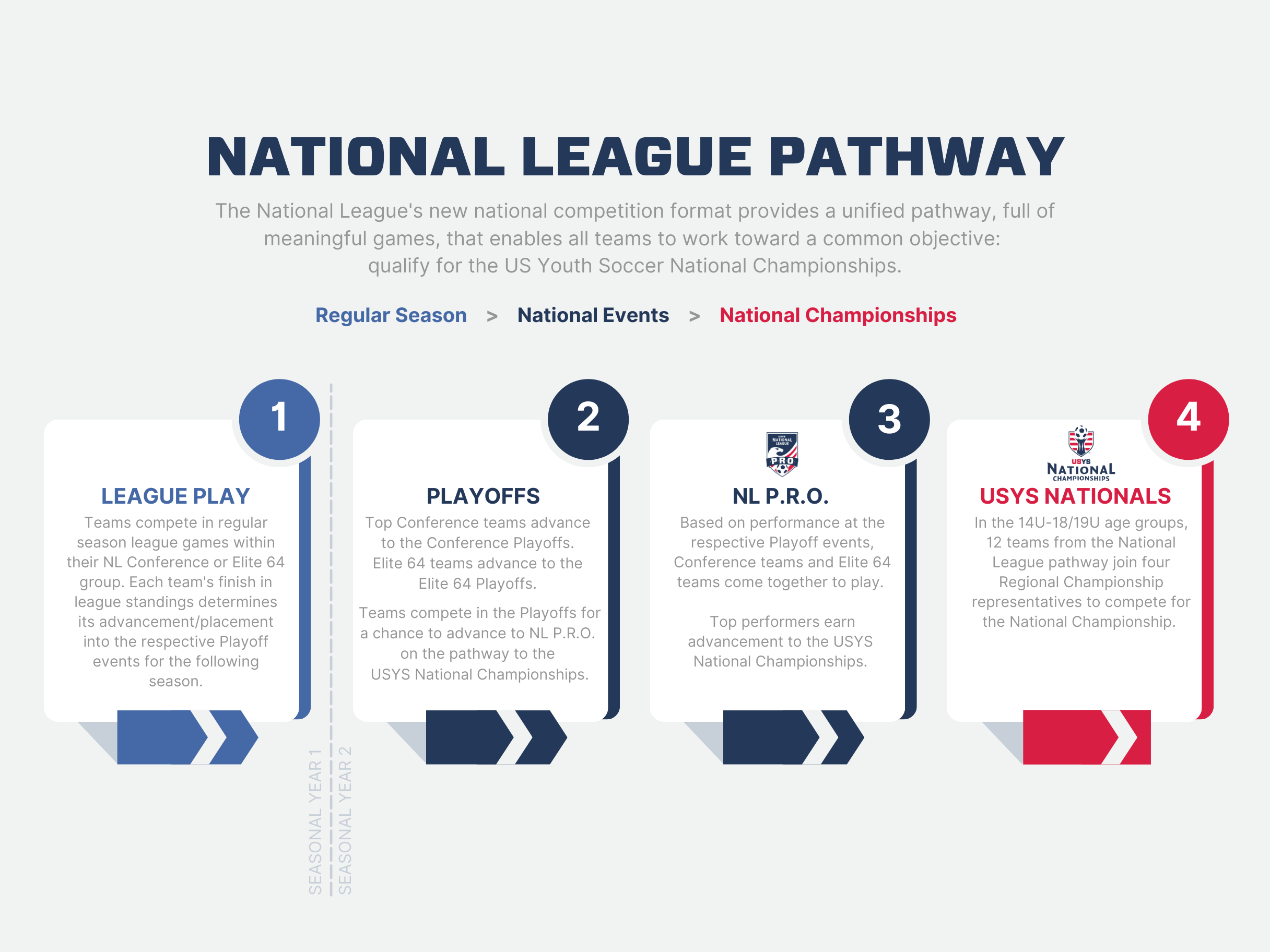The image is an informational poster titled "National League Pathway" in dark blue characters. It outlines the National League's new national competition format, which aims to provide a unified pathway filled with meaningful games, allowing all teams to work towards a common objective—qualifying for the U.S. Youth Soccer National Championships.

The poster is divided into four key sections, each highlighted in different colors, providing a step-by-step guide to the competition format:

1. **League Play**: Depicted in light blue, this section explains that teams compete in regular season games, with their standings determining placements for the next stage.
   
2. **Playoffs**: Also in blue, this part details that top conference teams advance to the conference playoffs. Success in the playoffs opens the possibility for teams to move forward to the NL Pro stage.
   
3. **NL Pro**: In a slightly darker blue, this section indicates that based on performance in playoff events, both conference and elite 64 teams come together to compete. Top performers in this stage earn advancement to the USYS National Championships.
   
4. **USYS Nationals**: Marked in red, this final stage describes that in the age groups 14U, 18, and 19U, twelve teams from the National League Pathway join four regional championship representatives to compete for the National Championship.

Overall, the poster serves as a detailed guide illustrating the progression from local league play to potentially competing for a national title, providing clear instructions and goals at each step of the pathway.